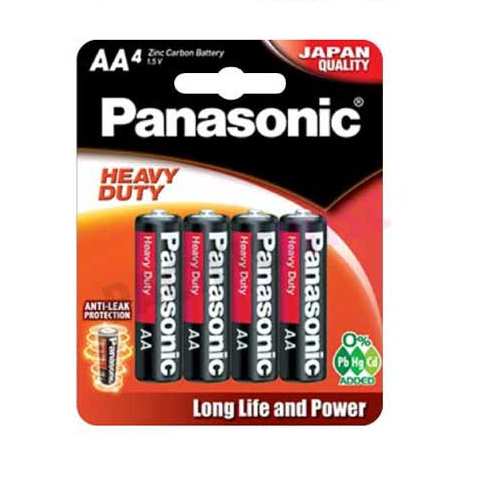A detailed image caption could be:

"This image showcases a pack of four Panasonic AA zinc-carbon batteries, known for their superior Japanese quality. Each battery is labeled 'Panasonic heavy-duty' and features '2A' or 'AA' prominently. The packaging includes a dynamic design with a swirling graphic of the battery on one side, symbolizing energy and movement. Additionally, the batteries offer anti-leak protection. To the left, there are three green circles marked with '0%' along with the chemical symbols 'PB', 'HG', and 'CD', indicating the batteries are free from lead, mercury, and cadmium. At the bottom of the packaging, an orange rectangle with white text proudly states 'Long Life and Power'. There is also a perforated hole at the top of the packaging for easy display on store hooks."